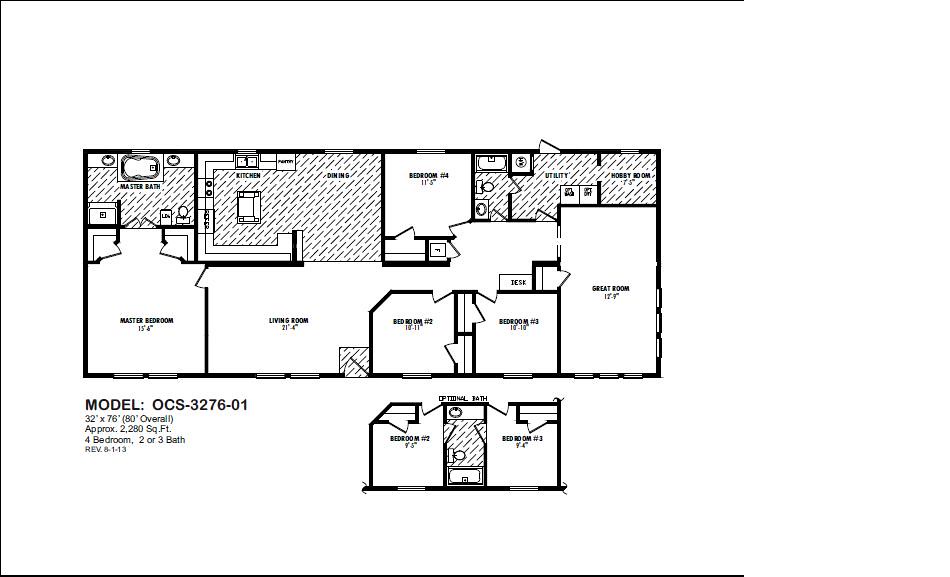This detailed floor plan depicts a four-bedroom home with the option of two or three bathrooms, identified as Model OCS-3276-01. The plan measures 32 feet by 76 feet, with an overall length of 80 feet, and encompasses approximately 2,280 square feet. This version is dated revision 8-1-13.

In the bottom left corner of the plan, textual information about the model is provided. The master bedroom, located on the very left, measures 15 feet 4 inches and features an adjoining master bathroom at its top. Adjacent to the master bedroom on the right is a spacious living room measuring 21 feet 4 inches in length.

Directly above the living room, the kitchen is positioned, complete with a standalone island in the center and configured in a C-shape layout with a range on the left-hand side. To the right of the kitchen is a dining area. Adjacent to the dining area on the right lies a bedroom measuring 11 feet 5 inches.

Below this bedroom is the second bedroom, sized 10 feet by 11 feet. To the right of this bedroom is the third bedroom, which measures 10 feet by 10 feet. Further to the right is a versatile Great Room, which measures 12 feet by 9 feet.

An alternate floor plan is presented below the main layout, which includes an optional third bathroom that is shared between bedroom numbers two and three.

In the top right section of the plan, a hobby room can be found. To its left is a utility room, and further left, a bathroom.

The floor plan offers a detailed and comprehensive view of a thoughtfully designed home layout, accommodating a variety of needs and preferences.